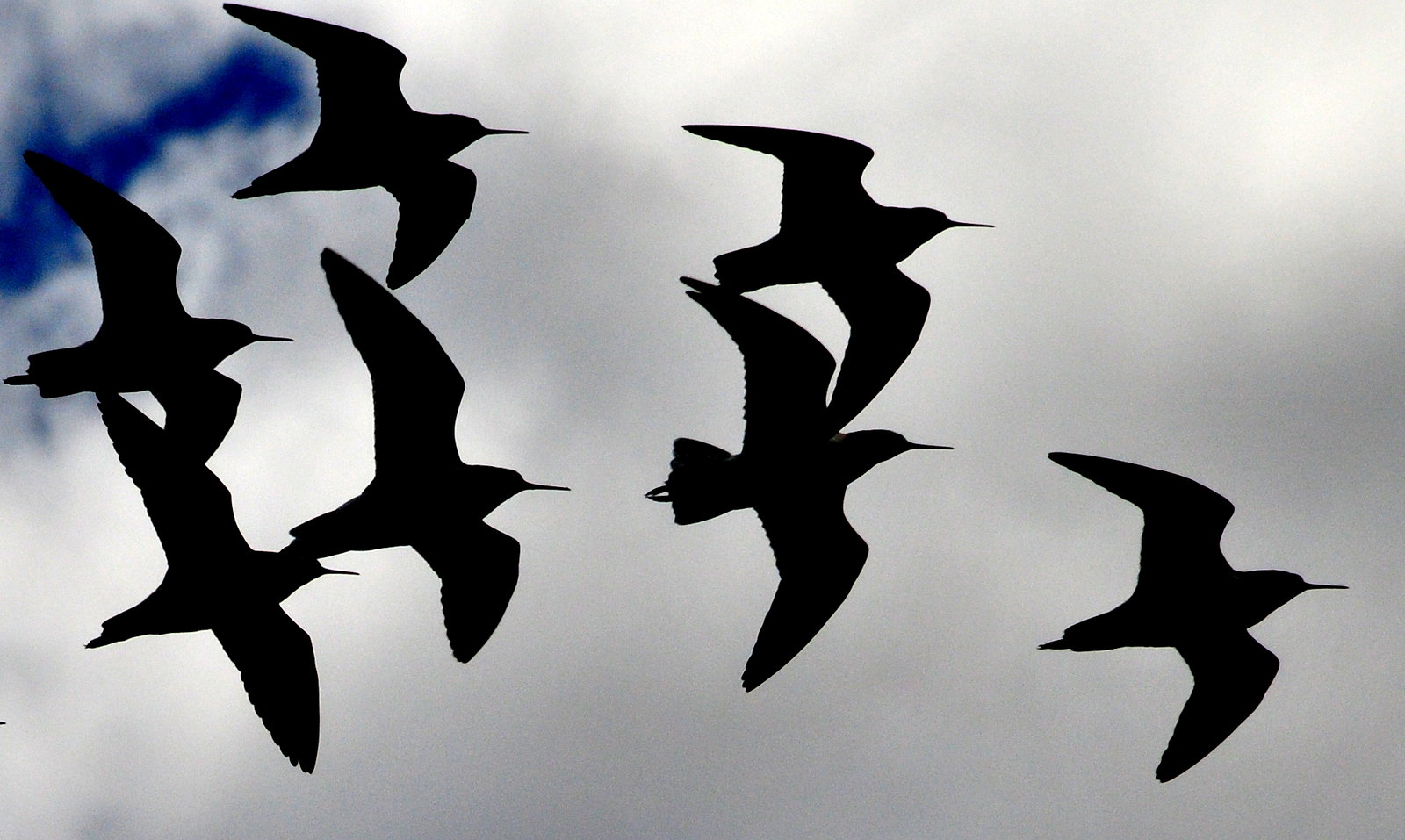In this daytime color photograph taken outdoors, an aerial view captures a striking scene of seven black birds in flight against a mostly cloudy sky with hints of deep blue peeking through in the upper left corner, suggesting a pretty day. The photographer stands below, pointing the camera straight up to emphasize the birds as the main focus. The birds, appearing as black silhouettes, all fly in formation towards the right. Details of their pointed bills and outstretched wings are visible, creating dynamic silhouettes against a backdrop of big white clouds with gray undertones. One bird is ahead at the bottom right, followed by a staggered formation of two pairs and another pair trailing behind. Some birds exhibit serrated wingtips and tails, adding to the intricate details captured in this moment.